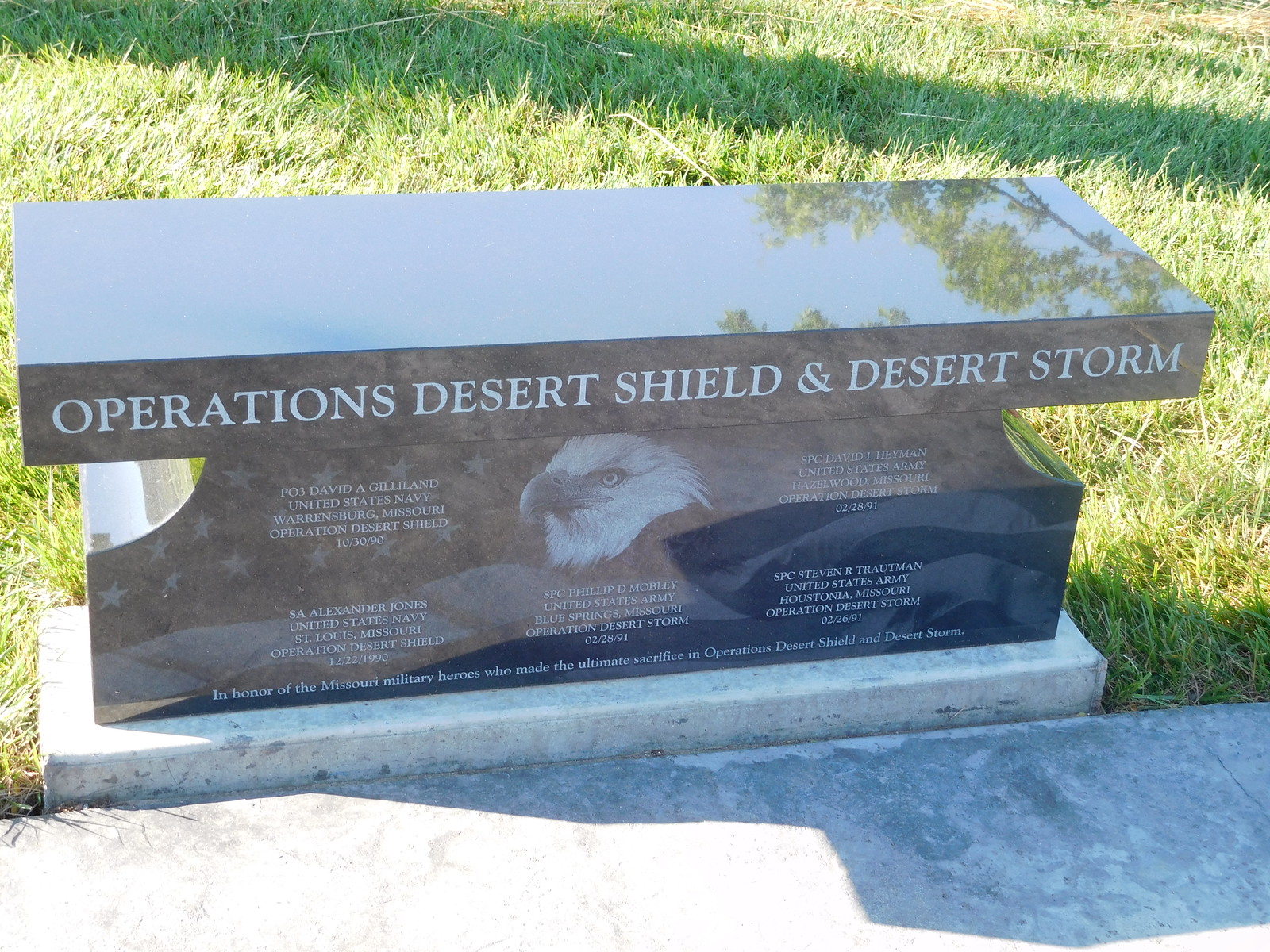This image depicts a memorial made from shiny, dark gray or black granite, standing on a flat stone base, with a flat top that reflects the surrounding scenery and sunlight. The memorial, reminiscent of a bench due to its size and flat top, honors Missouri military personnel who sacrificed their lives in Operations Desert Shield and Desert Storm. In the center of the memorial, an etched image features a bald eagle in front of an American flag. Engraved at the top in white letters are the words "Operations Desert Shield and Desert Storm." Below, several lines of text list the names of the fallen service members along with their ranks, branches of service, hometowns, and dates of death. Specifically mentioned are PO3 David A. Jillian from Warrensburg, Missouri, SA Alexander Jones from St. Louis, Missouri, SPC Philip D. Mobley from Blue Springs, Missouri, SPC David L. Hayman from Hazelwood, Missouri, and SPC Stephen R. Troutman from Houstonia, Missouri. At the bottom of the memorial, an inscription reads "In honor of the Missouri military heroes who made the ultimate sacrifice in Operations Desert Shield and Desert Storm." The background features green grass, with the image likely taken from the perspective of someone standing a few feet away, looking slightly downward. The sunny day casts light that causes shadows and reflections on the memorial’s surface.